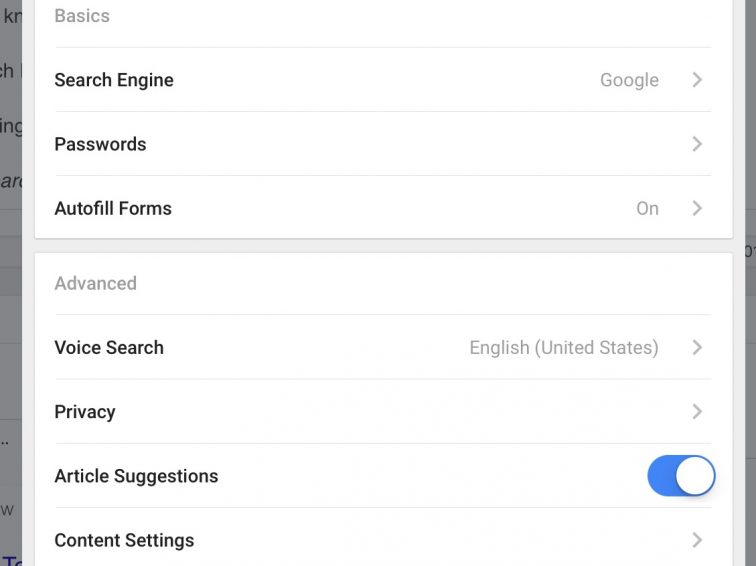The image is a detailed informational graphic presented in a square format with a multi-layered border. The outer edge features a thick dark gray border, which is broader on the left side compared to the right. This border transitions into a lighter gray strip that encapsulates the core content, which is set against a white background.

Within the white central section, the information is organized into clearly demarcated sections, each separated by thin lines resembling those on wide-lined paper. The first section starts with the label "Basics" in gray, followed by "Search Engine" in black text. Below this, the term "Google" with a forward arrow appears in gray text.

The next block within the same white section is labeled "Passwords" in black, followed by another forward arrow. Adjacent to this is the text "Autofill Forms" in black, marked as "On" with a forward arrow next to it.

The next major section is headlined "Advanced" in gray. Under this heading, "Voice Search" appears in black text, with "English (United States)" followed by a forward arrow to the right. The subsequent options include "Privacy" in black with a forward arrow, "Article Suggestions" in black marked as "On," and "Content Settings" accompanied by another forward arrow.

The overall layout is structured to offer a clear hierarchy and easy navigation through various settings, distinguished by alternating text colors and sectioning lines.